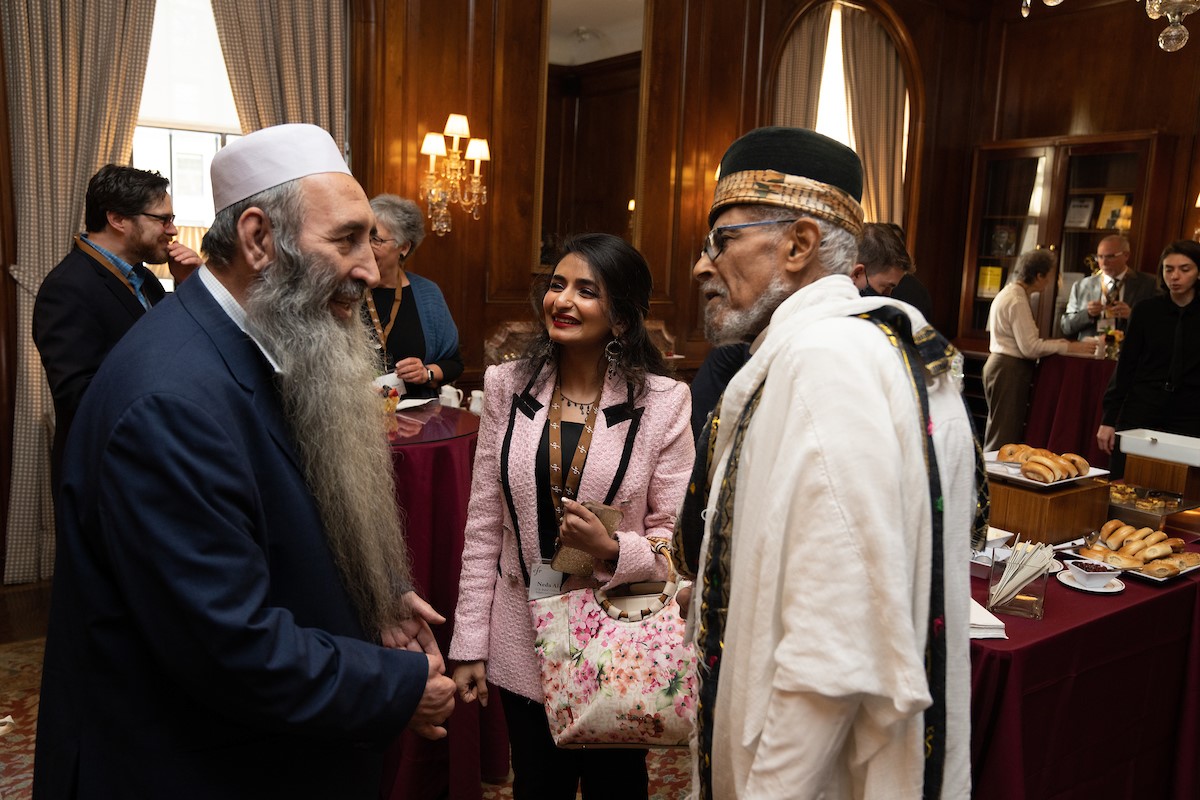In this photo, there is an indoor gathering, possibly in a hotel or banquet hall, featuring an assortment of bagels on elevated trays on a table. The centerpiece of the image is a scene involving three primary subjects. At the center is a Middle Eastern woman wearing a pink blazer and carrying a floral purse, engaged in conversation with two older men who seem to be religious officials. The man on the left, notable for his long grey beard extending below his chest, is smiling and dressed in a blue suit with a traditional white Middle Eastern hat. The man on the right, with a shorter beard, grey hair, and glasses, is dressed in predominantly white traditional attire with black decorations and a black hat. The setting includes windows with white and grey curtains, and a unique light fixture on the wall composed of three small lamps arranged in a triangular formation. Other people are in the background, adding to the lively atmosphere.